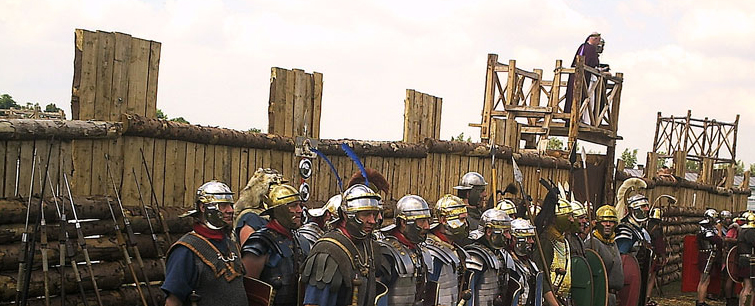The photograph captures a detailed scene of a Roman army reenactment set against a vivid outdoor backdrop. In the foreground, an array of Roman soldiers is lined up, dressed in varying styles of armor — silver plates, chain mail, and leather — all wearing authentic Roman helmets. They are armed with spears, swords, and shields, portraying the diverse equipment of a historical Roman legion. These soldiers stand before a wooden wall approximately eight to ten feet tall, featuring battlements and small pockets. On a wooden podium, around ten feet high near the center-right, two figures are prominently visible — one dressed in purple robes, likely representing a general, overseeing the scene. The photograph is angled from the left, capturing the soldiers from a side perspective, which adds depth to the composition. The background showcases tips of trees against a bright sky dotted with thick, white clouds, indicating a fair weather day. Additional wooden structures are also present, including an empty stand on the far right, enhancing the complexity and authenticity of the reenactment setting.